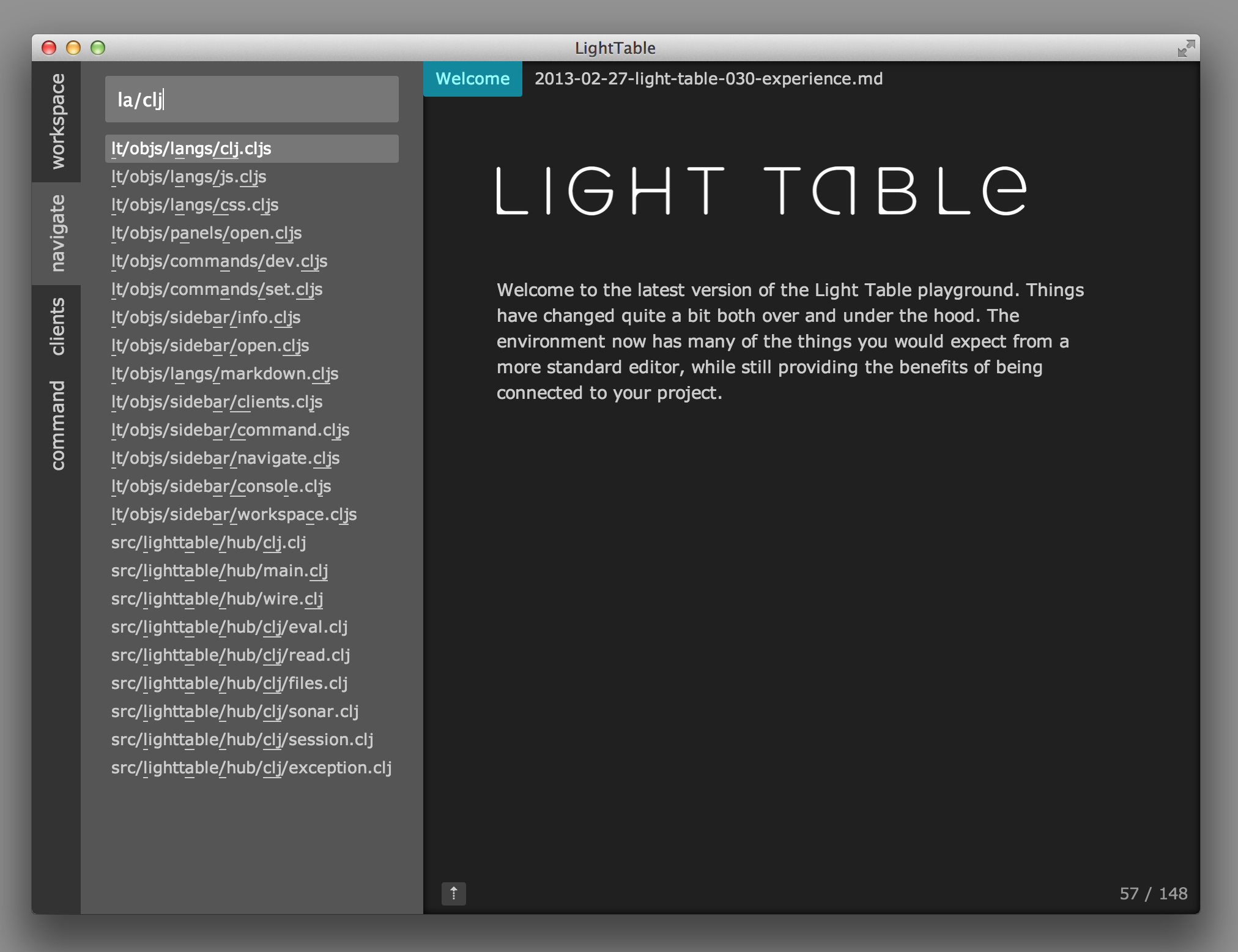This image is a detailed screenshot of an integrated development environment (IDE) called "Light Table," likely taken on a Mac computer due to the presence of the distinctive red, yellow, and green control buttons for closing, minimizing, and expanding the window at the top left corner. The interface features a vertical menu on the left side with options labeled "Command," "Clients," "Navigate," and "Workspace." The user has clicked on the "Navigate" tab, which opens a vertical pane with a dark gray background against the IDE’s overall black background. This pane displays what appear to be file destinations, with the top entry being highlighted and labeled "la/CLJ."

In the main section to the right, the title "Light Table" is displayed in an interesting font. Beneath this, there is a message in a small sans-serif white font that reads: "Welcome to the latest version of the Light Table playground. Things have changed quite a bit over and under the hood. The environment now has many of the things you would expect from a more standard editor while still providing the benefits of being connected to your provider." Finally, the bottom right corner of the screen features two numbers, "57" and "148," in small gray text.